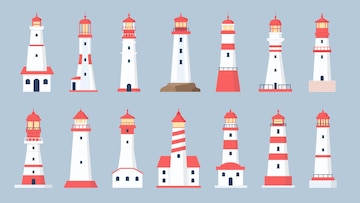This image is a small rectangular drawing, approximately two inches wide and one inch tall, featuring 14 lighthouses arranged in two rows against a blue, almost periwinkle background. Each row has seven distinct lighthouses. All the lighthouses share a white body with red accents, and their lights at the top glow a yellowish hue. The designs show a variety of structures: some are tall and conical, while others include homes or buildings at their bases. The patterns vary, with some lighthouses adorned with horizontal or diagonal stripes, while others remain plain. Additionally, some lighthouses feature black fences, doors, and windows. Although unified by their color scheme, none of the lighthouse designs repeat, showcasing an array of architectural styles.